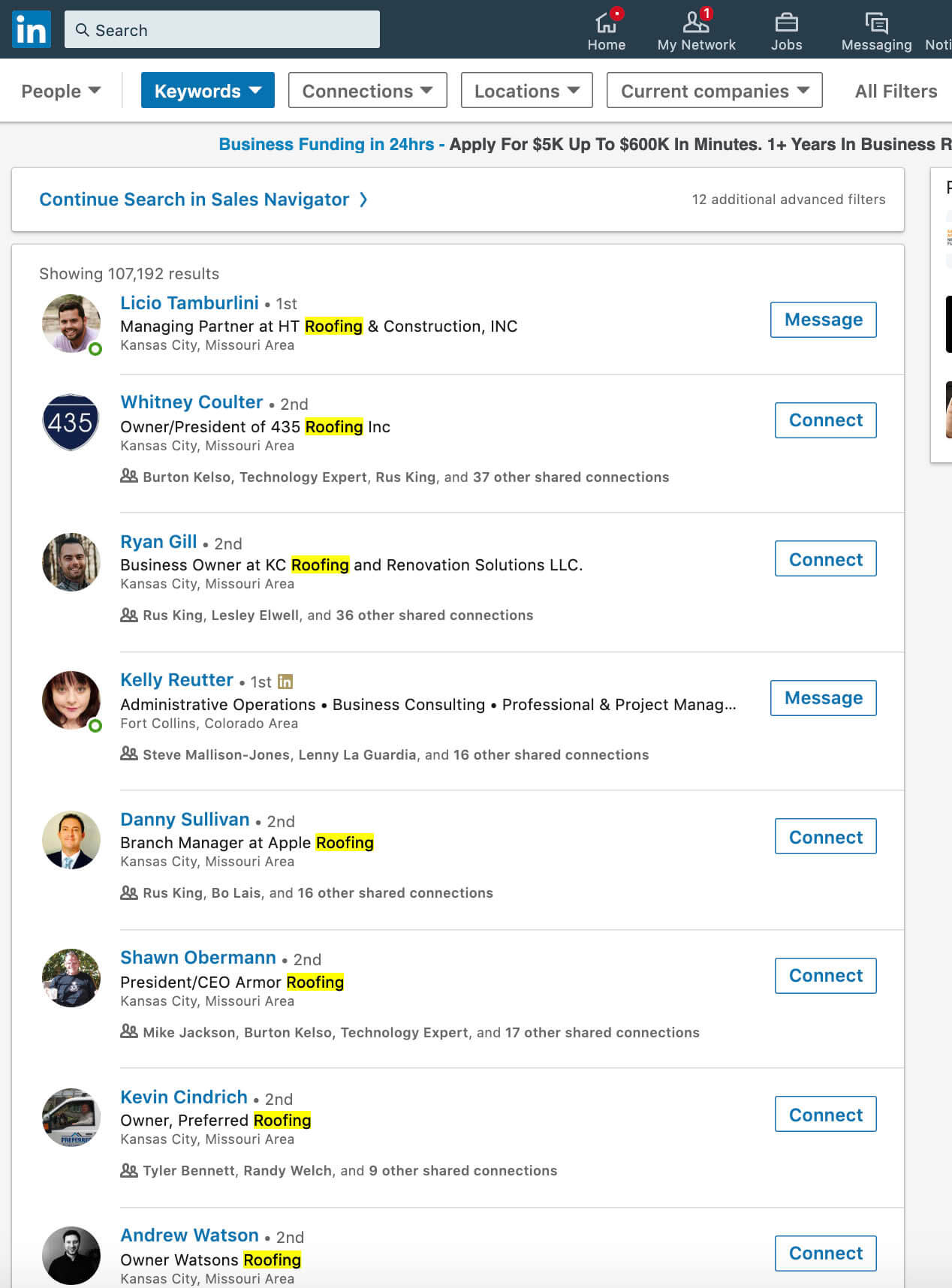This is a detailed screenshot of a LinkedIn interface. 

At the top left, the iconic LinkedIn logo is displayed—a blue square featuring the white lowercase letters "in." Adjacent to it on a darker blue top ribbon, there's a white search box equipped with a magnifying glass icon. To the right of this search box, navigational options include "Home," "My Network," "Jobs," and "Messaging," all in white text accompanied by respective icons. Both "Home" and "My Network" display red notification circles indicating pending updates.

Below this ribbon, there's an advanced search area featuring various filters. This white section allows users to refine their searches using boxes labeled "People," "Keywords," "Connections," "Locations," and "Current Companies." Notably, the "Keywords" filter is highlighted in blue.

Further down, there is an informational section promoting business funding options, with text in blue and black advertising quick loan applications ranging from $5,000 to $600,000. Below this advertising area, a white banner with blue text provides navigation links labeled "Continue Search" and "Sales Navigator."

The majority of the screen is dominated by a large white box divided into nine sections, each representing a different LinkedIn user's profile. Each section includes:
- A profile picture on the left.
- The user's name displayed in blue.
- Job titles and descriptions in black text.
- A location listed beneath the job description in gray text.

To the right of each profile section, there are interactive buttons outlined in blue with blue text, either "Message" or "Connect." Specifically, the first and fourth profiles have "Message" buttons, while the remaining profiles feature "Connect" buttons.

The job description for each individual, except the fourth person, includes the word "roofing," which is highlighted in yellow for emphasis.